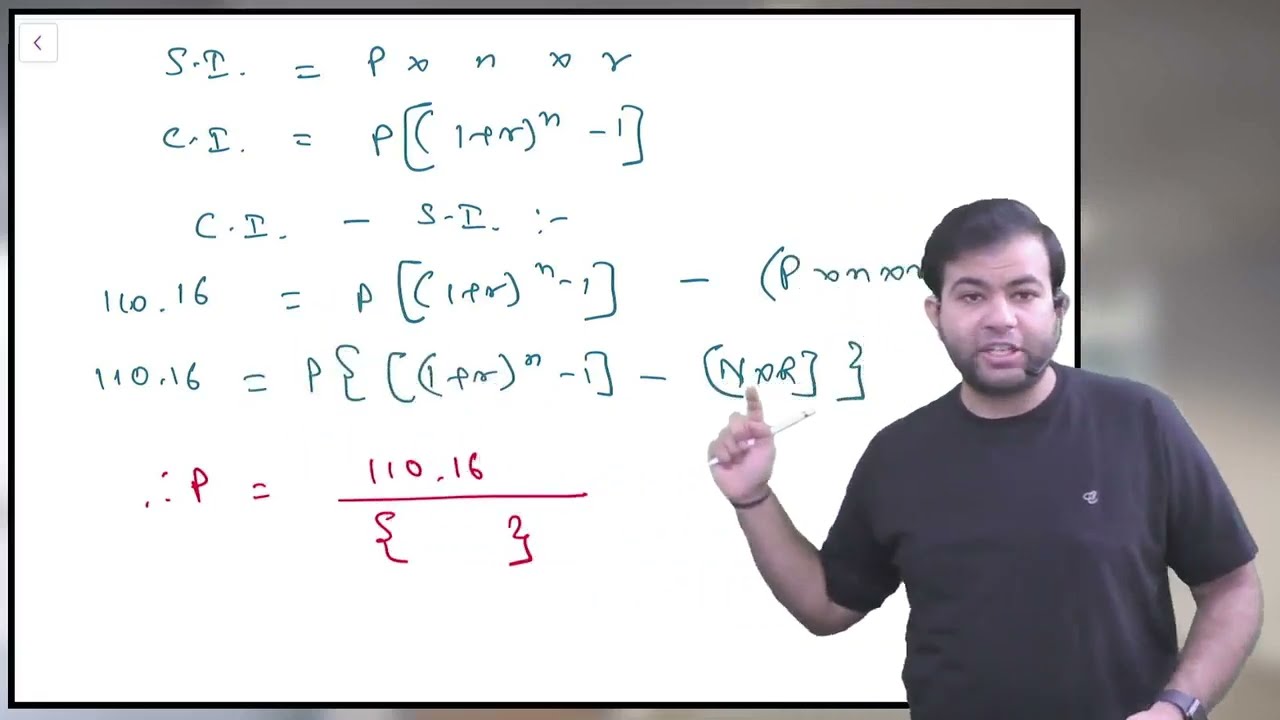The image depicts a man standing in front of a white digital display board, outlined in black, covered with complex mathematical computations and symbolic notations in both green and red. The markings include various figures in brackets, letters like 'P', 'S', 'I', and an infinity symbol, suggesting advanced mathematics or coding topics. The man, positioned on the right-hand side near the center of the image, has short black hair, a stubbly beard, and appears to be speaking as his mouth is open. He wears a black t-shirt with a small white emblem on the left chest and has a smartwatch on his right wrist. His right arm is raised, pointing with his index finger towards the board while holding a white marker, ostensibly to write on the digital display. His left arm hangs by his side. Additionally, he seems to be wearing a headset with a microphone on the left side of his face, indicating that he might be conducting a virtual teaching session, reflected by the slightly off-color tint typical of webcam footage. The background to the right of the image is blurry, adding to the focus on the man and the whiteboard.